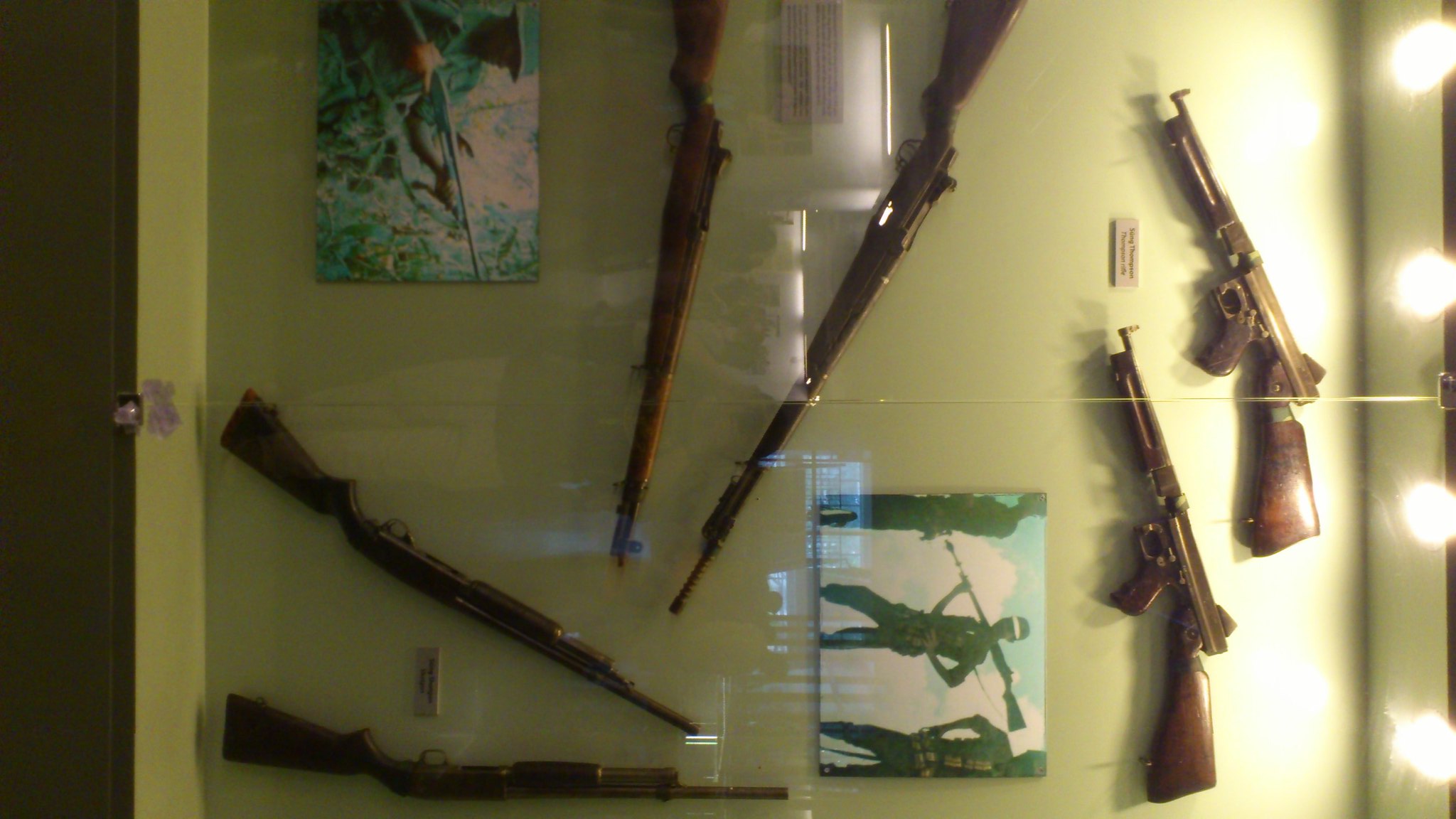In this colour photograph, we observe a glass-encased, somewhat blurry display of historical rifles, displayed in an indoor setting. The image is skewed sideways, necessitating a 180-degree rotation to view it correctly, with the original top positioned on the right and the bottom on the left due to improper phone orientation during capture. In the background, towards the upper right corner, a vertical alignment of four round lights shines onto the display, casting vague reflections off the glass. 

On the left side of the display, there's a brown door with a metallic knob. Just above this door, there's an abstract painting using hues of blue and green. Within the display case, a total of six rifles are arranged. Two rifles are placed diagonally downwards on the left side, two larger rifles are positioned upwards and slightly to the left in the middle section, and two more rifles are on the lower left corner. Small plaques, likely containing information about the rifles, are interspersed between them but are illegible due to blurriness.

Embedded among the rifles, on the lower middle portion of the photograph, is a smaller rectangular image of a painting depicting three gunmen against a white backdrop with a blue sky, appearing as if they are in green military uniforms. This image is oddly placed on its side, rotated so you have to tilt your head to the right to view it properly. In addition, there are reflections of what appear to be metallic elements in the glass, including a round object with a purple rectangle and a narrow tube seen between the middle rifles. Further, another image of a man in military uniform holding a rifle appears below the first image, contributing to the militaristic theme of the exhibit, which seems indicative of a World War II or Vietnam War period.